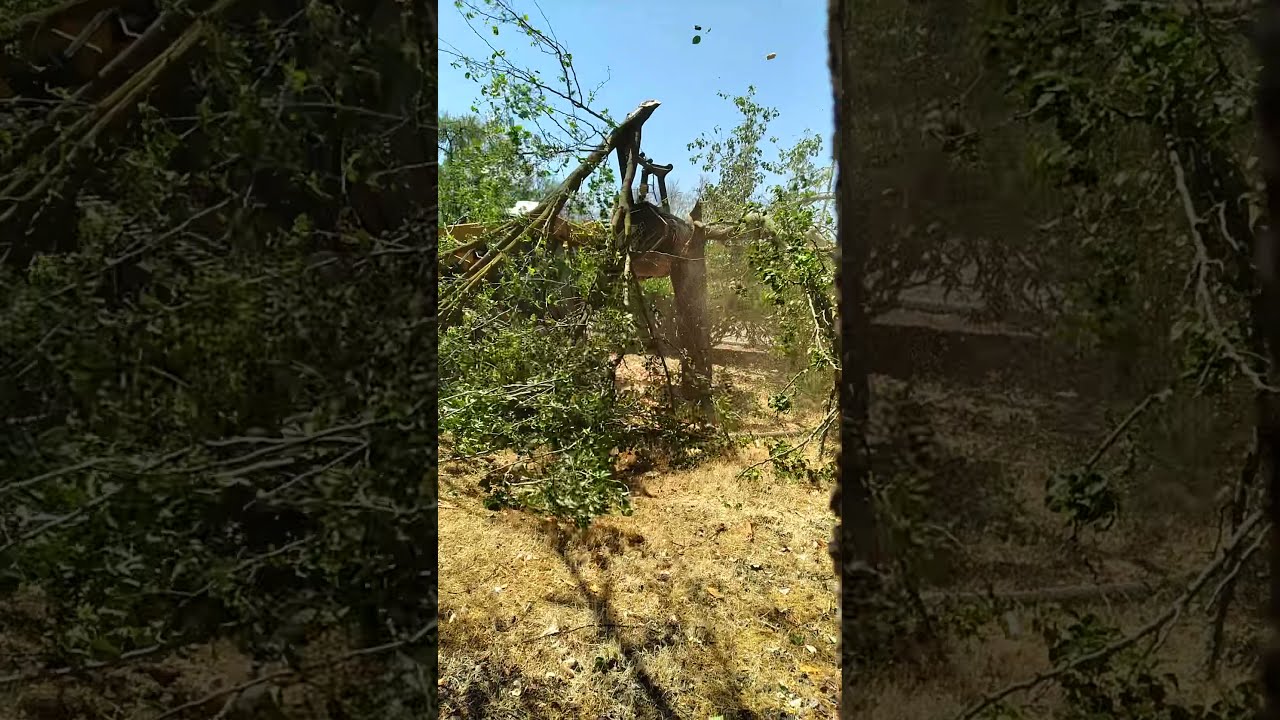The image portrays an outdoor scene under a clear blue sky, devoid of clouds, with sunlight illuminating the area. The central focus is a large tree that appears to have snapped and fallen, lying flat across a patch of tan-brown, dead grass. The fallen tree's branches, still laden with green leaves, are scattered across the ground, mingled with other tree trunks and branches leaning against or lying beside the fallen giant. A visible tree stump stands upright, hinting at where the tree might have once stood. 

Surrounding the main scene are two smaller, darker-framed images—one on the left, the other on the right. These side images seem to be fragments or closer views of the middle picture, emphasizing the presence of bushes and more tree debris. In the background, a wooden fence can be glimpsed, suggesting an enclosed area. Despite the chaotic aftermath of the tree's fall, the bright daylight underscores every detail, casting no direct shadows but illuminating the remnants vividly.